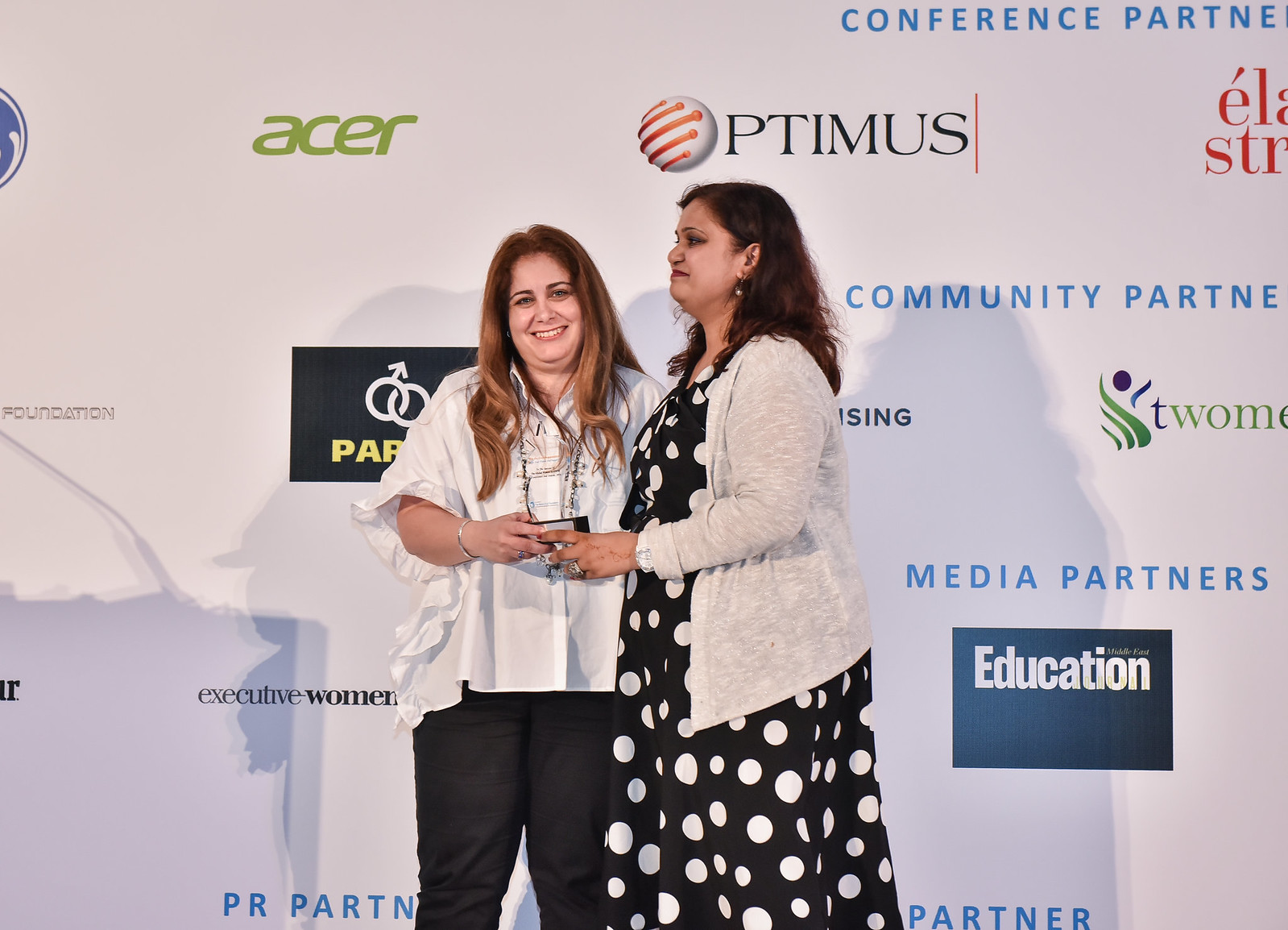In the image, two women are centered against a colorful backdrop featuring advertising from various companies, such as Acer, Mobile East Education, and Executive Women. The background wall displays a mixture of orange, light green, black, yellow, and blue hues.

The woman on the left, who is facing the camera, has long brown hair and fair skin. She is smiling and wears a white short-sleeved baggy shirt with black pants. In her right hand, she holds an award. Beside her, the second woman, seen in side profile, has dark curly hair and wears a gray sweater over a black and white polka dot dress. She appears to be making a cringy face. With her left hand, she also holds the same award.

The setting suggests a conference or event where awards are being presented, indicated by the backdrop that lists conference and media partners.